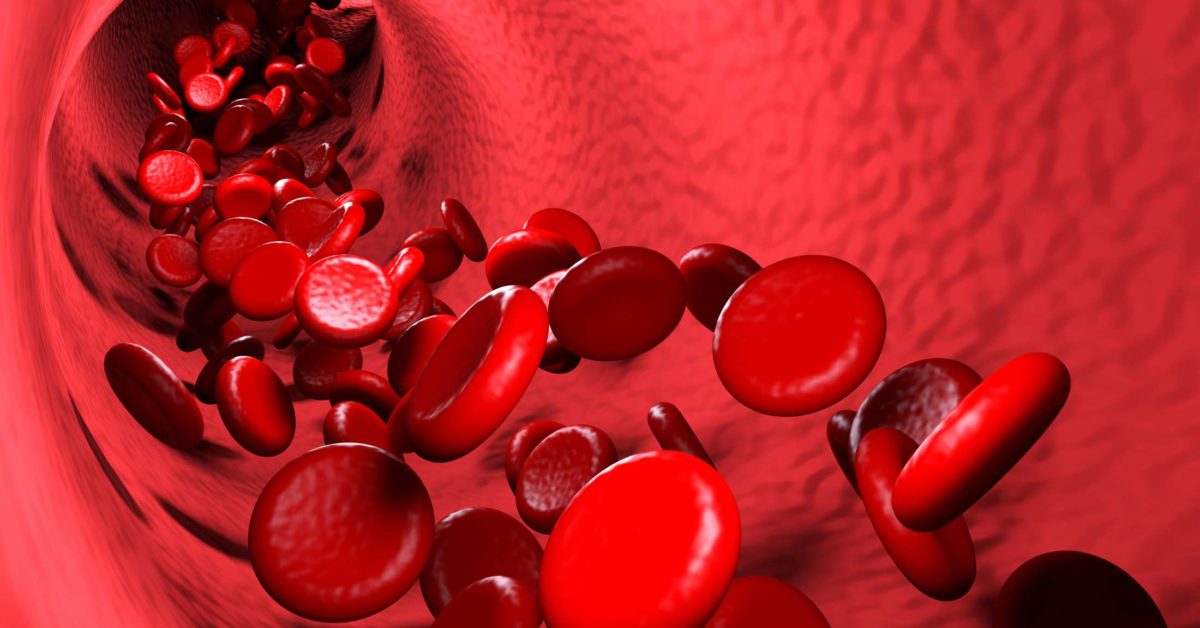The image is a detailed and vivid 3D representation of the interior of a vein or artery, with rough, textured red walls that create a tunnel-like structure. Down this tunnel, which stretches from the upper left to the lower right of the image, flows a dense cluster of at least a hundred red blood cells. The blood cells are depicted as flat, rounded disks, similar to frisbees with a smooth surface on one side and a slight indentation on the other. The cells vary in tone from bright to darker red but maintain a consistent red color overall. As the cells move closer to the viewer, they appear larger, showcasing the 3D aspect of the illustration. This striking visualization captures the dynamic, crowded nature of red blood cells traveling through the bloodstream.